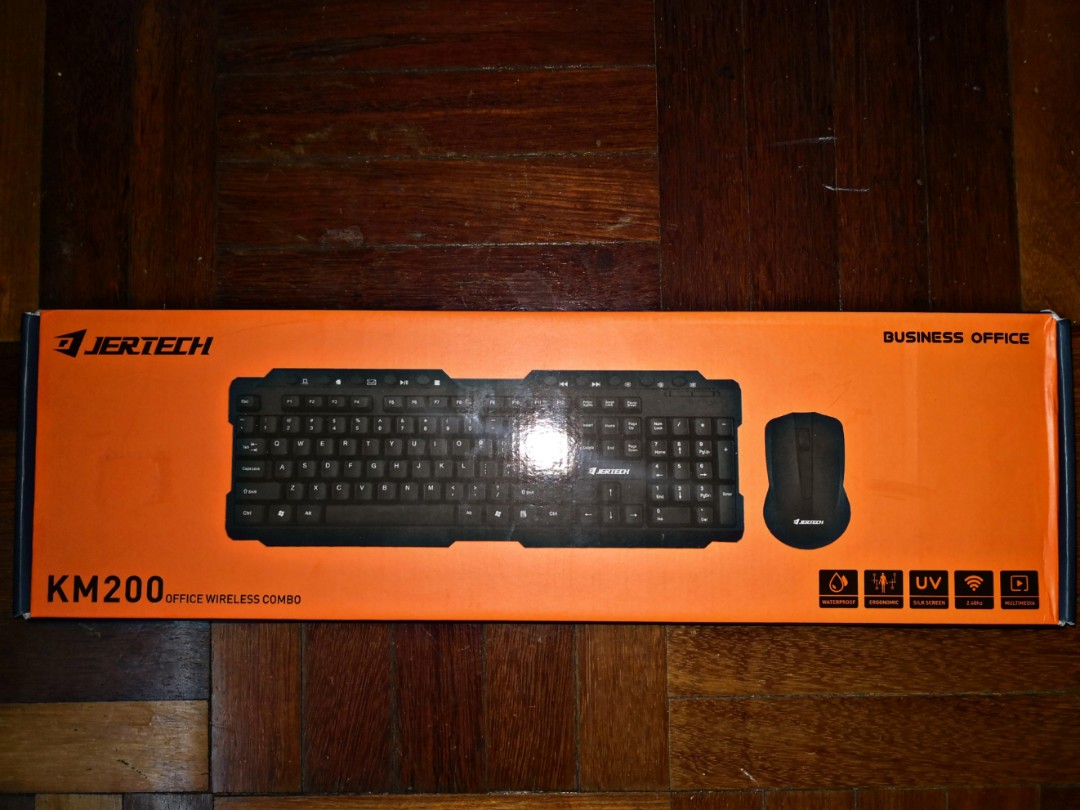This image features a dark brown, semi-reflective wooden surface. It is unclear whether the surface is a table or a floor. Illuminated by a light source from above, there is a warm glow reflecting off the surface. Central to the composition is a rectangular-shaped orange box with black sides on the left and right edges. The top left corner of the box is branded with "Jertech," followed by the text "KM 200 Office Wireless Combo." The box prominently displays a black keyboard and a black mouse in its center. The overhead light creates a noticeable round glare on the box. In the top right corner of the box, the phrase "Business Office" is printed, while the bottom right corner of the box features five small square labels or symbols, each containing different text that is not clearly legible.